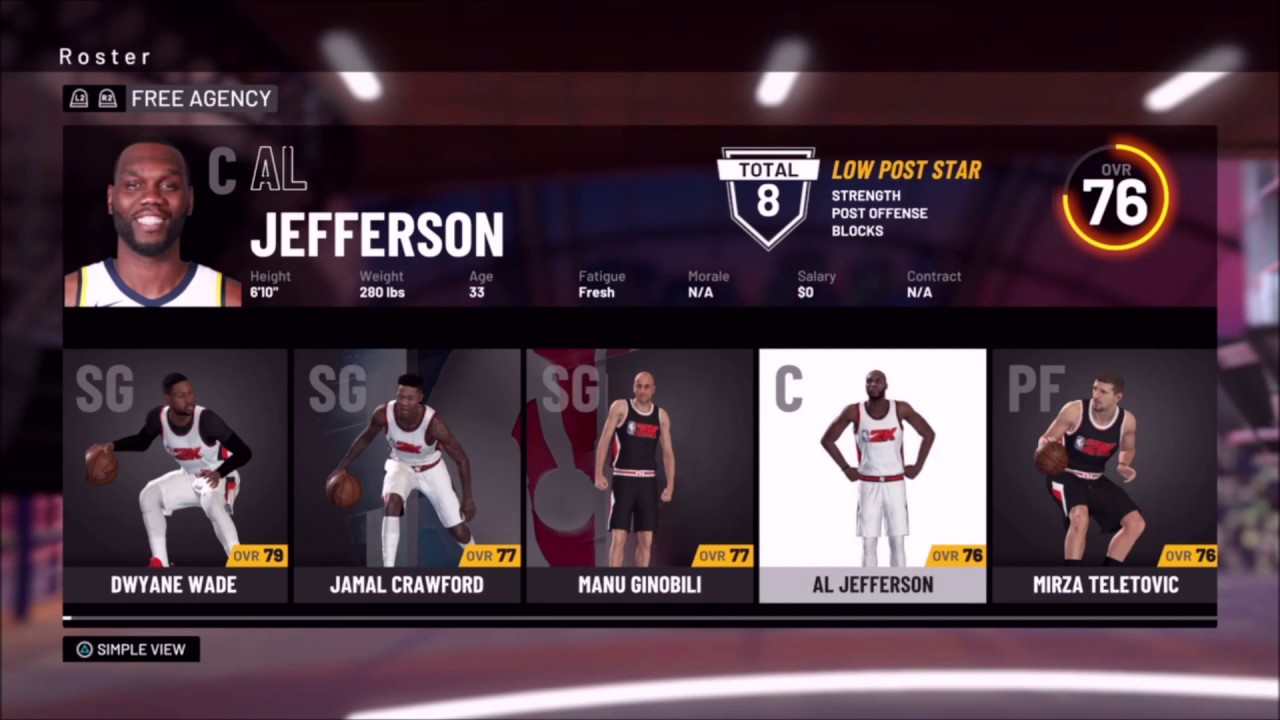This is a detailed descriptive caption for the image described:

The image appears to be a screenshot from an NBA-themed video game, likely NBA 2K, focusing on the game's "Roster" and "Free Agency" sections. The background, which has a blurred visual reminiscent of a locker room or basketball hall, features long tubular ceiling lights and various crates on the left side, along with a window on the right side partially blurred to keep the focus on the foreground.

In the top left corner, the word "Roster" appears, followed by "Free Agency" in a black rectangle accompanied by two icons. Dominating the center of the screen is an African American player named Al Jefferson, wearing a white jersey with yellow side stripes and blue accents, complete with a Nike swoosh. The player’s details are listed as follows: height of 6'10", weight of 280 pounds, age of 33, fatigue status as fresh, morale listed as NA, a salary of $0, and his contract status also shown as NA.

In the top right corner, a shield symbol shows the number 8. Just below this, "Low Post Star" is highlighted in yellow text, and strengths in "Post Defense" and "Blocks" are indicated in white text. Al Jefferson's overall rating is displayed prominently as 76, surrounded by a yellow glow in a circular bar chart, signifying a 76% fill with the abbreviation "OVR" and the number 76 in white text.

There are five player images below this section: Dwyane Wade with an overall rating of 79, Jamal Crawford with a 77 rating, Manu Ginobili with a 77 rating, Al Jefferson with a 76 rating, and Mirza Teletovic also rated at 76. Each player is depicted in action or posing for the camera.

Additionally, a small box at the bottom right of the screen labeled "Simple View" suggests an option to switch display modes for the roster information.